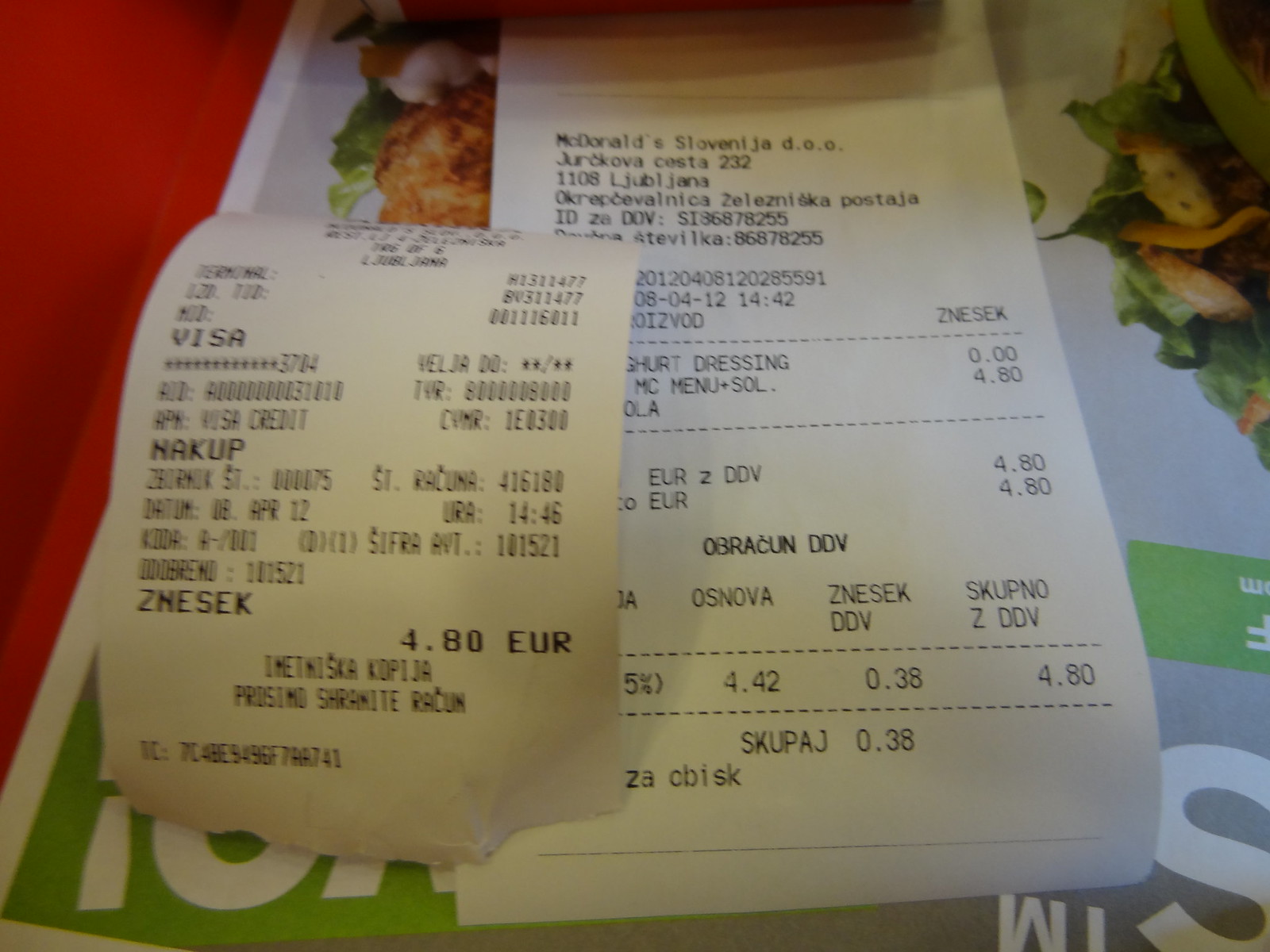The image depicts two receipts positioned side by side, with the one on the right clearly marked as being from McDonald's. The McDonald's receipt appears to include items such as yogurt dressing among other entries, though some parts are unreadable. In another language, the receipt mentions a payment made via Visa, with the last four digits of the card being displayed. Notably, the figure "$4.80" can be seen on the receipt.

Beneath the receipts, there is a bread tray serving as a liner on which some chicken and a mix of green and orange vegetables are arranged. The overall composition suggests a combination of commercial fast food items and fresh produce, creating a juxtaposition of different types of meal components.